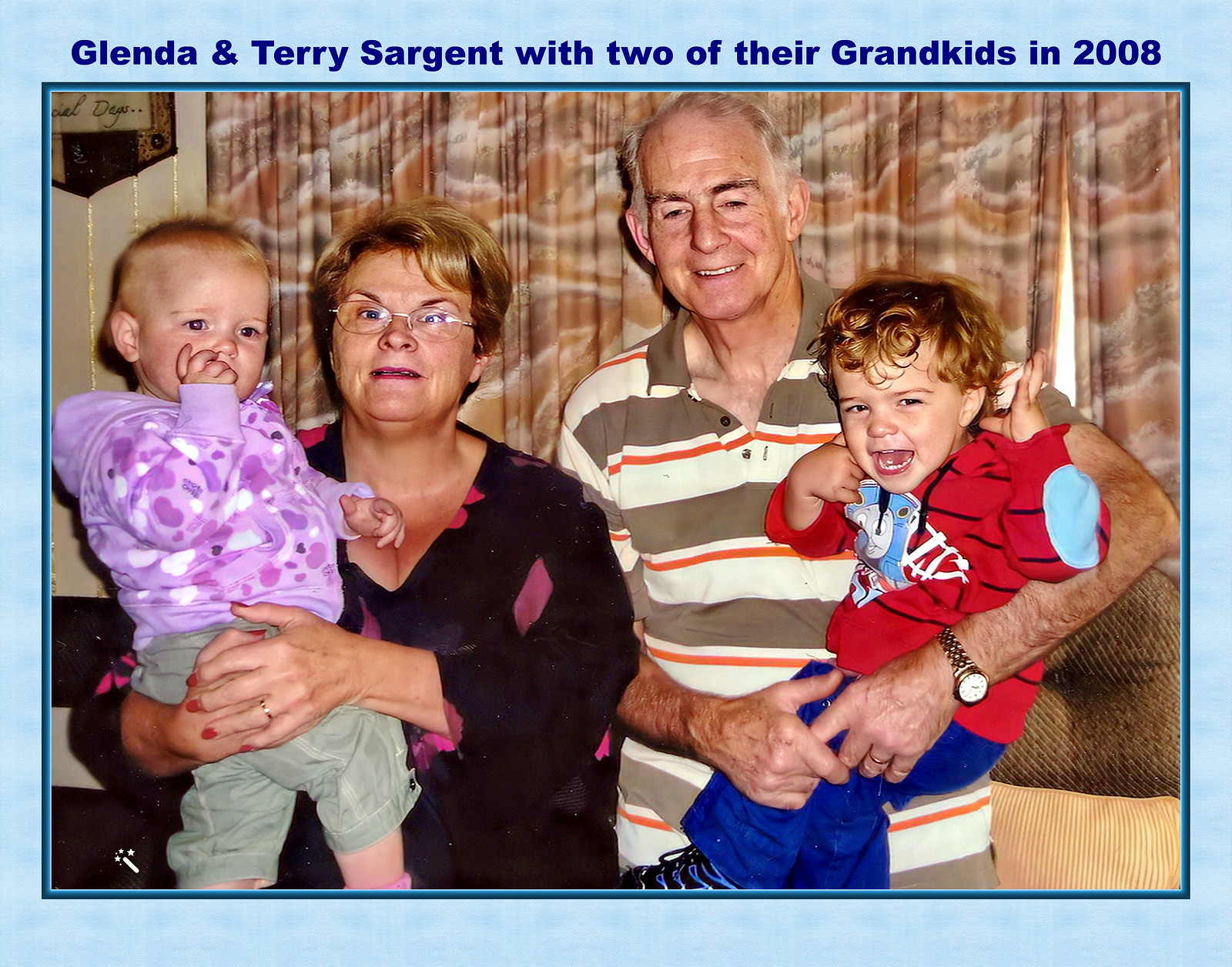The photograph, bordered by a blue line with a darker blue outline, features Glenda and Terry Sargent with two of their grandchildren in 2008. Above the image, it is labeled with their names and the year. Glenda, on the left, is a Caucasian woman wearing glasses and a dark blouse with pink accents, holding a young girl with a purple hoodie and gray pants. Glenda also sports red nails and a ring on her left hand. Her light brown hair frames a surprised expression as she looks towards the camera. Terry, on the right, is an elderly Caucasian man with thinning gray hair, sporting a watch on his left wrist. He is dressed in a light shirt with dark brown and red stripes, holding a young boy who is wearing a red shirt and blue pants. The boy, with semi-curly light brown hair, appears to be crying. Both children are fairly young, with the girl having very short light brown hair and green capris, while the boy is also wearing sneakers.